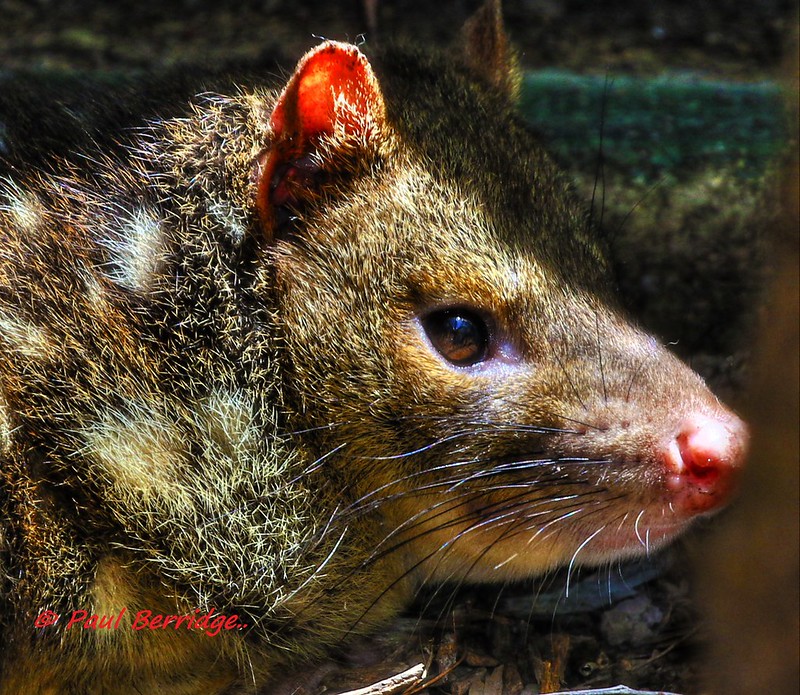A close-up, sunlit image of a marsupial-like animal, potentially from greater Australasia. The creature bears a close resemblance to a possum, characterized by mixed brown, gray, white, and black fur. Its most prominent features include short, round, semi-translucent ears, a light pink nose, long black whiskers, and expressive brown eyes. The animal's elongated snout and larger ears set it apart from a typical squirrel. In the bottom-left corner of the image, the name "Paul Berridge" is displayed in red italicized font, possibly indicating the photographer. The outdoor setting appears natural, with a dark, woodsy, and forested background.